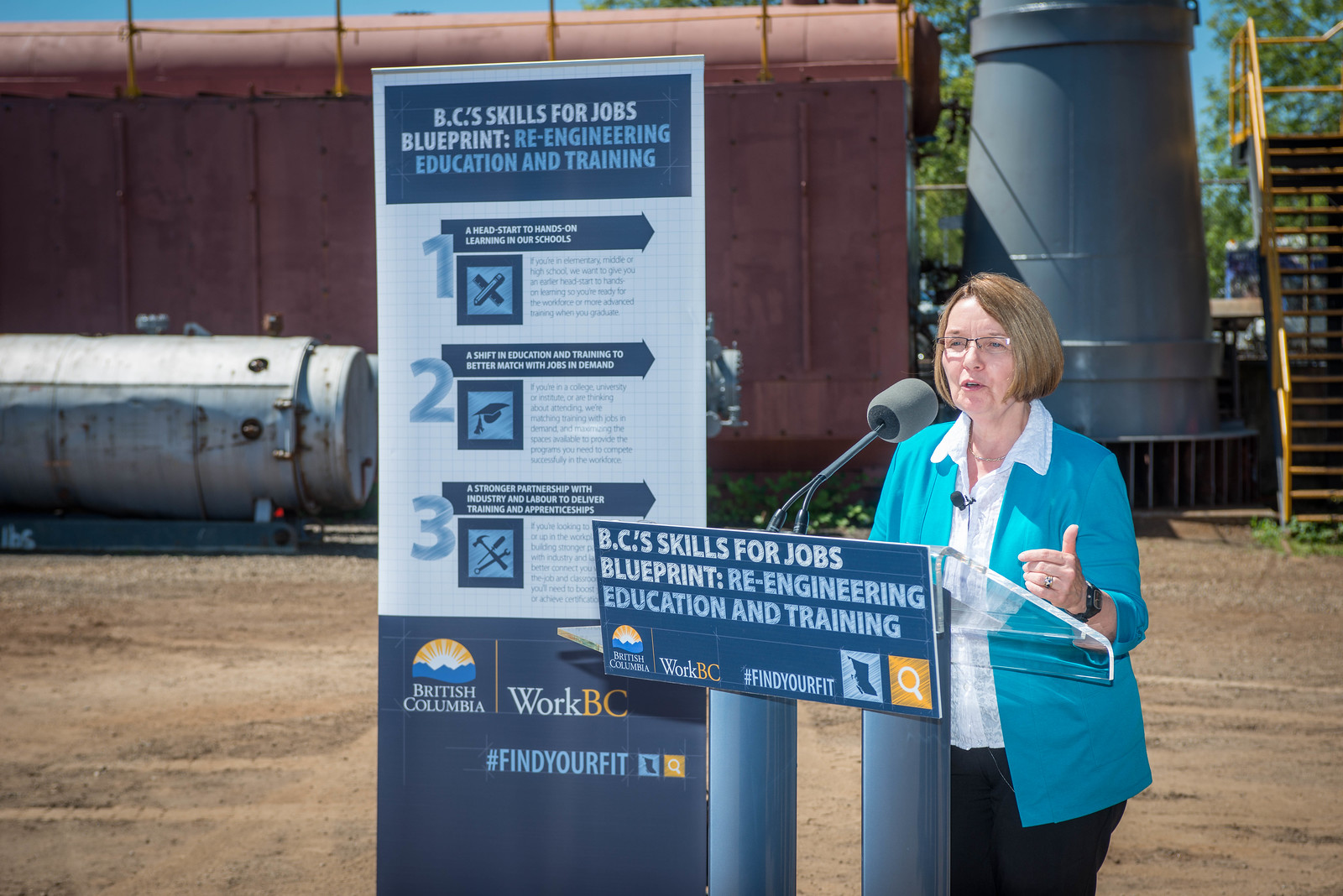The image depicts a woman with short brown hair and Caucasian skin standing behind a podium, which is angled about three-quarters to the left. She is dressed in a bright blue jacket over a white collared shirt and brown pants. The podium prominently displays the words "BC's Skills for Jobs Blueprint: Re-engineering Education and Training" against a blue background, with the text in light and slightly darker sky blue. Logos in orange and blue appear across the bottom of the podium.

To her left, there is a large sign that shares the same title "BC's Skills for Jobs Blueprint: Re-engineering Education and Training" at the top on a blue background. Beneath that, on a white background, is a numbered 1-2-3 list detailing the steps: 
1. Head start in hands-on learning in our schools.
2. Education and training better matched with jobs in demand.
3. Stronger partnerships with industry and labor to deliver apprenticeships.

The woman appears to be speaking at an outdoor event, with light brown dirt underfoot and machinery as well as industrial-looking buildings made of gray or brown metals visible in the background. Additional details on the sign include the British Columbia logo, phrases like "Work BC," "Find Your Fit," and graphical elements such as a map and a magnifying glass.